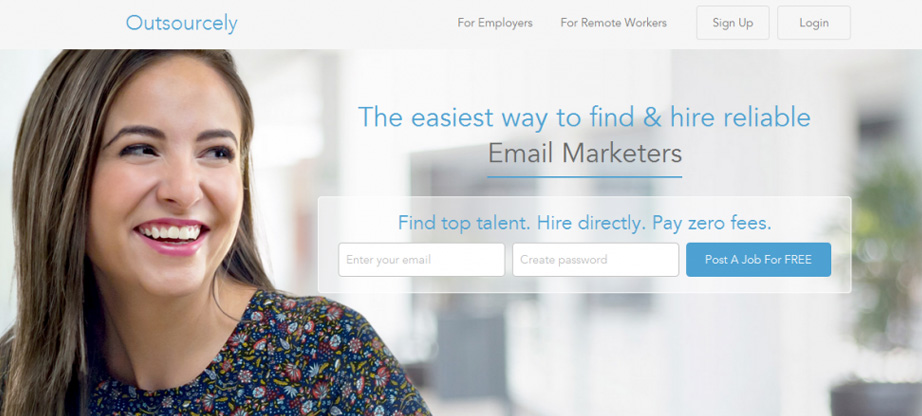The webpage for Outsourcely is presented with a clean and professional interface. At the top of the page, in a sleek gray box, the word "Outsourcely" appears in a vibrant aqua color. Adjacent to this, there are navigation links labeled "For Employers" and "For Remote Workers," accompanied by "Sign Up" and "Log In" buttons. These elements are styled in lighter and darker shades of gray text, with the buttons featuring light gray borders and backgrounds.

Immediately below this section, there is an image of a woman on the left-hand side. She is dressed in a blue shirt adorned with a distinctive paisley and floral pattern in shades of blue, red, and yellow. She is smiling warmly, her bright red lipstick complementing her brown hair with blonde highlights. Her brown eyes are directed towards the text on the page, which reads "The easiest way to find and hire reliable email marketers." The phrase "The easiest way to find and hire reliable" is written in aqua blue, whereas "email marketers" is in dark gray, underlined with an aqua blue line.

Further down, within another light gray rectangle, key benefits are highlighted in aqua text: "Find Top Talent," "Hire Directly," and "Pay Zero Fees." Below these points, there is a faint gray text box inviting users to "Enter Your Email" and a password field labeled "Create Password," also in light gray text. Finally, a prominent "Post a Job for Free" button appears, styled in aqua with white text, with "Free" emphasized in all capital letters.